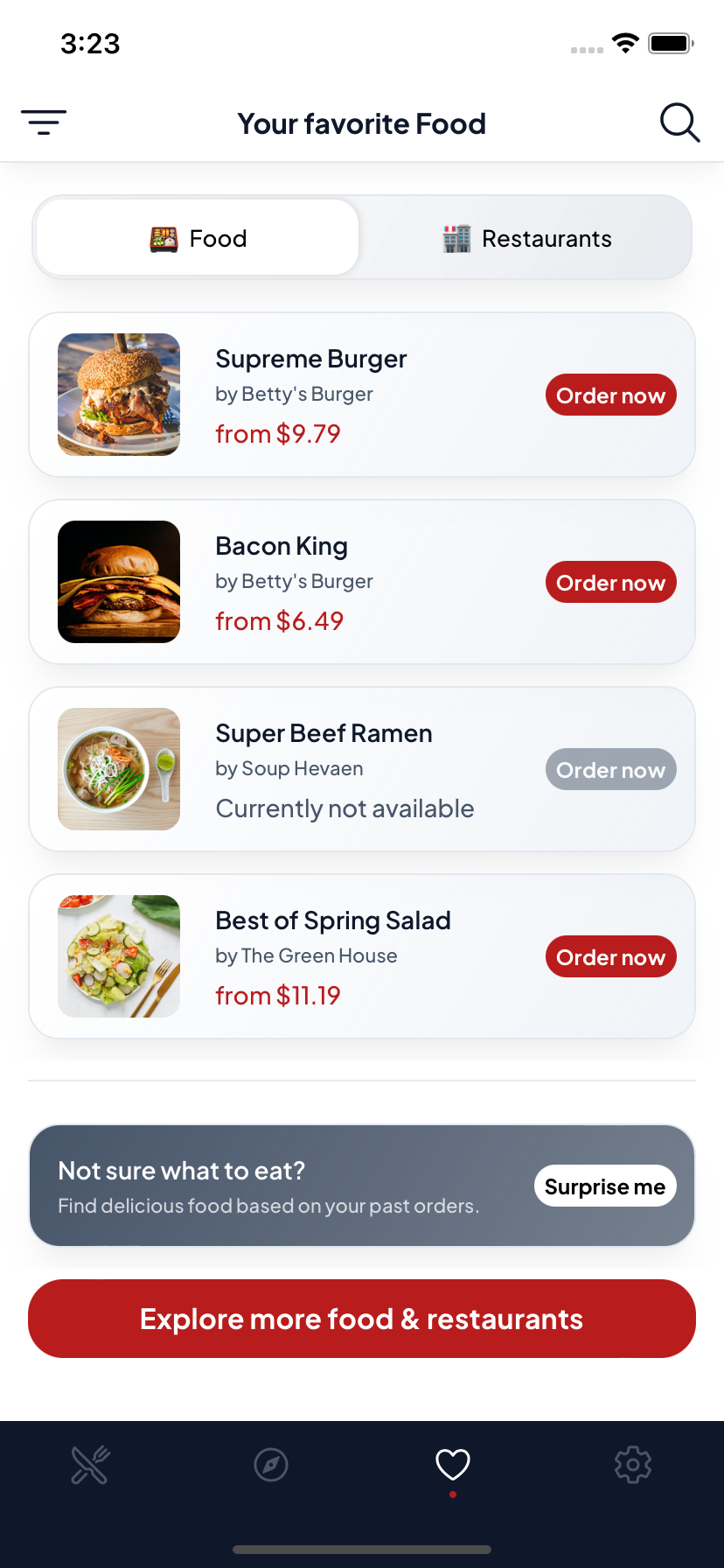This mobile-optimized web page appears to be a food ordering platform, offering a convenient browsing experience tailored for smartphone users. At the top of the page, users can see a heading that reads "Your Favorite Food," with options to filter what they are looking at via two tabs: "Food" and "Restaurants." The current view is filtered to display food directly.

Among the highlighted options, there is the "Supreme Burger" from "Buddy's Burger," priced starting at $9.79. Another item is the "Bacon King," also from "Buddy's Burger," starting at $6.49. However, the "Super Beef Ramen" from "House Heaven" is marked as not available. Additionally, there is "The Best of Spring Salad" from "The Greenhouse," starting at $11.19.

An intriguing feature below these offerings encourages users who are uncertain about what to eat. It states, "Not sure what to eat? Find delicious food based on your past orders," with a clickable "Surprise Me" button that would allow the website to curate recommendations tailored to the user's previous choices. There’s also an "Explore More Food and Restaurants" option, which presumably offers a broader selection influenced by the user’s order history.

The interface also includes a settings button at the bottom right corner, providing easy access to customizable options. The timestamp on the screenshot indicates that it is 3:23, though it is not clear if it is AM or PM.